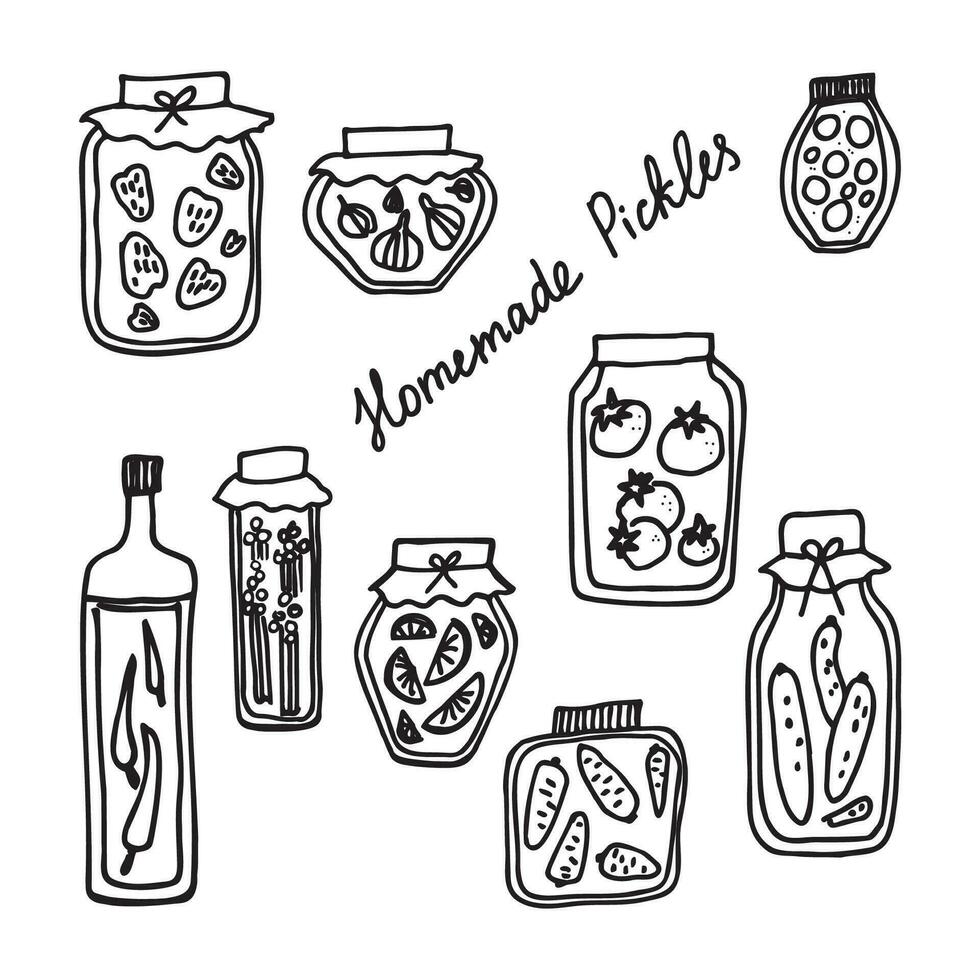The image is a detailed black and white sketch featuring numerous jars, bottles, and cans of varying shapes and sizes, all drawn with a black marker. Each container is intricately illustrated with different types of pickled items, prominently labeled with handwritten text that reads "Homemade Pickles" at the center, extending towards the top right. In the top left corner, a jar filled with pickled strawberries is depicted with a cloth tied with a bow covering its top. Other jars around the sketch show a variety of pickled produce: garlic, tomatoes, carrots, limes, lemons, oranges, chili peppers, artichokes, and slices of pickles. Some jars feature unique shapes like rectangular and square forms, and one bottle in the center right contains round pickles, suggesting it might also hold other vegetables. The consistent theme across the image showcases an array of homemade pickled vegetables and fruits, each container contributing to the artisanal and rustic charm of the composition.